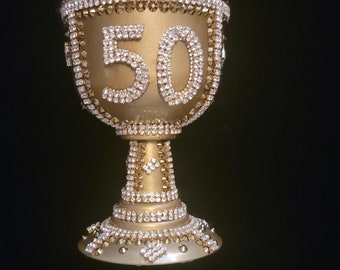The image features a centrally positioned gold trophy resembling a chalice against a completely black background, giving it a dramatic contrast. The trophy, which likely symbolizes a 50th celebration such as a birthday or anniversary, is adorned with an array of ornate clusters of sparkly rhinestones or imitation diamonds. The gemstones embellish the entire trophy, including a prominent '50' on the cup portion, crafted from white and gold gemstones. The trophy emits a slight glow, enhancing its regal appearance. The ornate design continues down the stem to the base, which is lighter in gold with a touch of silver at the very bottom, suggesting a metal construction. The simplicity of the background ensures that all attention is drawn to the detailed, sparkling centerpiece, with no other text or items in the frame.